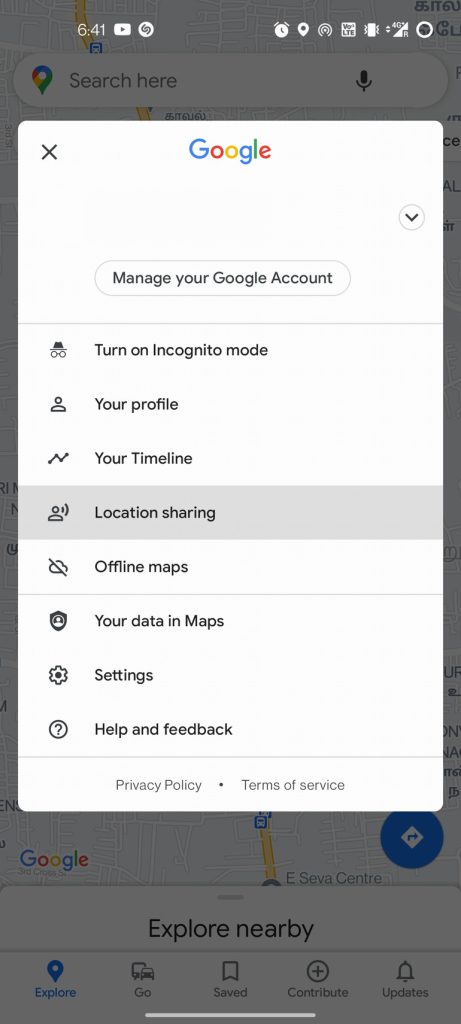This is a detailed screenshot of the Settings menu from the Google Maps app. At the top of the screen, the header reads "Google," followed by comprehensive options: "Manage your Google Account," "Turn on Incognito Mode," "Your Profile," "Your Timeline," "Location Sharing," "Offline Maps," "Your Data in Maps," "Settings," and "Help & Feedback." In the background, a bit of the Google Maps interface is visible. At the bottom of the screen, the text "Explore nearby" can be seen, along with five icons labeled: "Explore," "Go," "Saved," "Contribute," and "Updates." 

In the top left corner of the screen, the time is displayed as 6:41. Additionally, there are small icons for YouTube and Shazam, the music recognition app. Toward the right-hand side at the top, there are icons for an alarm, location, and a blue sharing icon. Further to the right are icons for mobile data, vibrate mode, and signal strength.